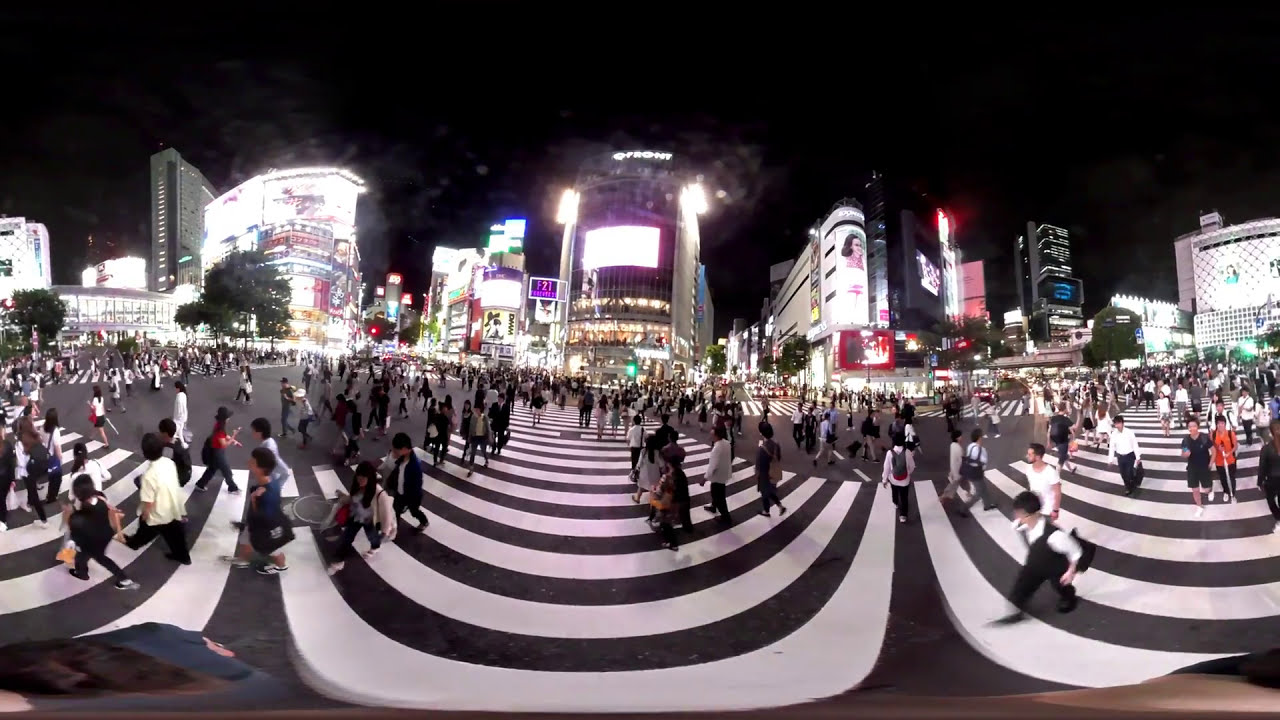This panoramic nighttime photograph, likely taken in a bustling Asian city such as Hong Kong, Beijing, or possibly Singapore, captures a lively, urban scene. In the foreground, a wide street features multiple crosswalks with bent, white, slashing lines arching like upside-down rainbows. Large numbers of people, predominantly of Asian descent, are seen crossing the street in various directions, creating a scene of dynamic movement and energy. 

The background showcases tall, illuminated buildings, suggesting commercial establishments like shops and restaurants, adorned with multicolored lights and advertisements reminiscent of a vibrant cityscape similar to Las Vegas. The sky above is an opaque, pitch-black expanse, intensifying the high contrast between the city's bright lights and the night. The color palette in the image includes shades of black, gray, white, as well as vibrant hues of purple, pink, red, orange, blue, and green. This rich array of colors highlights the neon-lit ambiance typical of major urban settings in Asia.